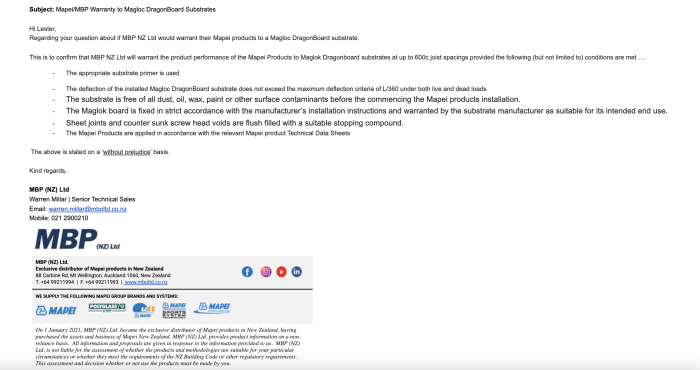In this image, there is a text document detailing a warranty confirmation from MBP NZ Limited. The subjects of the document revolve around Maple Dub MBG and MBP products and their compatibility with Maglog Dragon Board substrates. It begins with an introductory note, "Hi, Atlefstar," addressing a query regarding whether MBP NZ Limited would warrant their MagPi products when used with Maglog Dragon Board Substrates. The message clearly states that MBP NZ Limited will guarantee the performance of Maple products on Maglog Dragon Board Substrates at temperatures up to 600°C, provided specific conditions are met. These conditions include:

1. The use of an appropriate substrate primer.
2. Ensuring that the deflection of the installed Maglog Dragon Board Substrates does not exceed the maximum deflection criteria of L360 under both live and dead loads.

Additionally, the document mentions that joist spacing specifications must be adhered to, although the provided text does not detail them fully. The overall tone of the message is authoritative and aims to provide clarity on warranty coverage and installation requirements.